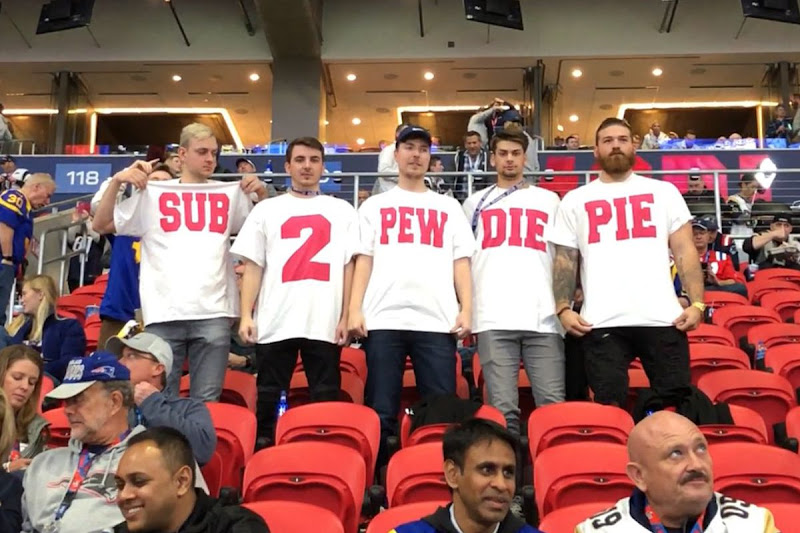In this vibrant image taken at a football stadium, a sea of spectators dressed in various colors fills the background, with many sporting blue and red jerseys. Red seats are prevalent throughout the stadium, adding to the lively atmosphere. The central focus of the image is a group of five young men standing amidst the crowd, each wearing a white t-shirt. The t-shirts together spell out a message: the first shirt prominently displays "sub," the second one reads "to," followed by "PewDiePie" on the next three shirts. The individual with the "sub" shirt is holding it high to make the text clearly visible. Behind them, rows of empty seats, a gate, and club seating are discernible, along with stadium lights and TV monitors above. This candid yet posed moment, aimed at showing support for PewDiePie's YouTube channel, captures the energy and camaraderie typical of a sporting event, possibly an outdoor football game given the context and the attire of the fans.